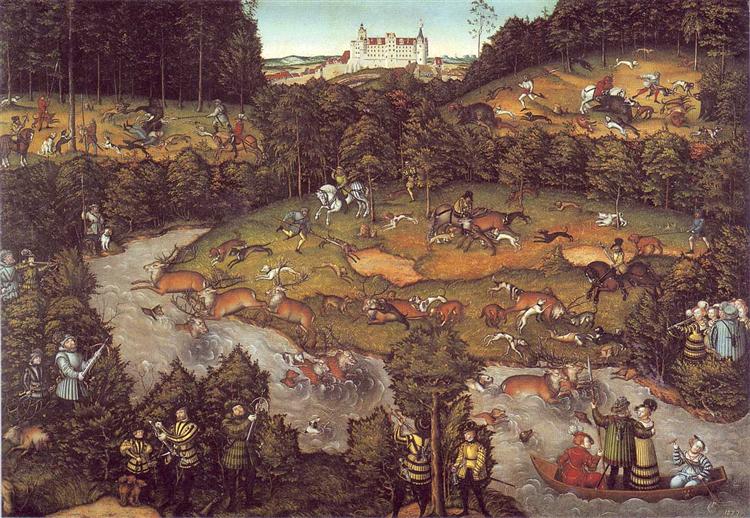This intricate painting evokes a sense of historical nostalgia, blending elements of playful artistry with a hunting scene from what seems to be a medieval or early Victorian era. Dominating the background, a grand white castle with a red roof stands majestically, overseeing the scene below. The focal point, however, is the lush, sprawling gardens and dense forest in the foreground, where autumn's touch is evident in the green and greyish foliage and imperfectly green grass.

The land is teeming with life and activity. Animals abound—deer leaping over water, cows dotting the landscape, and dogs running about—indicating a lively hunting scene. Nobles, adorned in ornate yellow and black striped outfits resembling bumblebees, participate in the hunt, some with crossbows, while the nobles near the river enjoy a leisurely boat ride, including three well-dressed women and a man in a long green coat.

Every portion of the painting vibrates with movement, from the playful behavior of animals and the strategic positioning of hunters to the serene presence of boats floating down the river, all weaving together a vivid tapestry of a royal hunt in an exquisitely picturesque and bustling medieval-like setting.